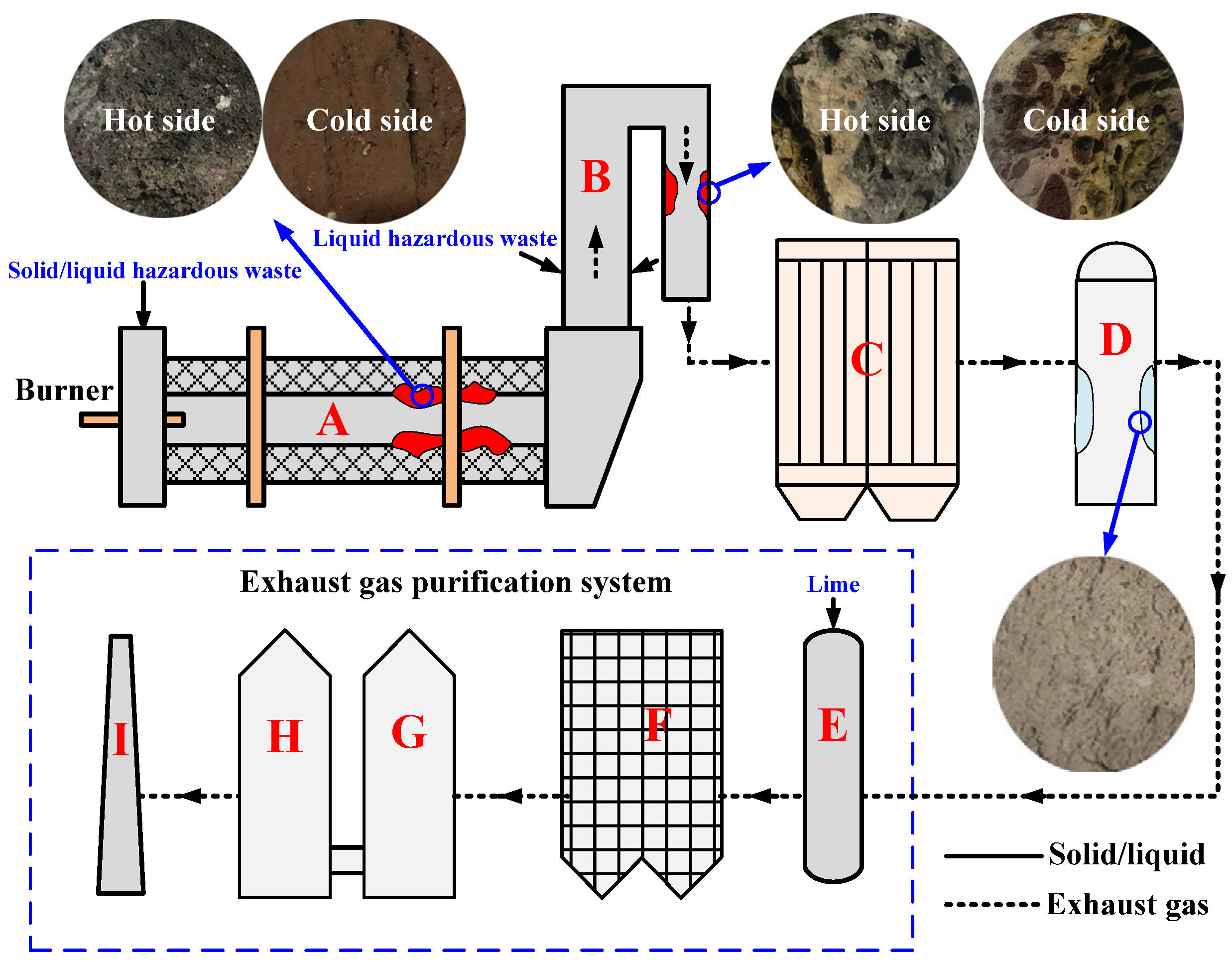This detailed diagram illustrates a waste incinerator system. The diagram is set in a rectangular, landscape view, clearly marking a "hot side" and a "cold side" at both the top left and top right corners. Key process components are represented by letters A through I, guiding the waste through various stages of the system.

Starting at the top left, the diagram depicts an input section labeled as "solid/liquid hazardous waste" which enters a burner denoted by a square. This burner opens into chevron-shaped pipes labeled Area A, filled with red material indicating the hot side. The waste then proceeds through several sequential processes: 

1. **Area A:** The burner labeled for solid/liquid hazardous waste connects to chevron pipes, moving the waste into the system.
2. **Section B:** A wedge-shaped item receives hazardous liquid waste, directing it upwards and along pipes.
3. **Section C:** Represented by two inverted Roman columns, this section collects the routed material through designated arrows.
4. **Section D:** Shaped like a bullet with components on either side, possibly indicating a conversion or reaction phase, it directs exhaust gases through dotted lines.
5. **Exhaust Gas Purification System:** Enclosed within a dashed blue box containing sections E through I, this system cleanses the exhaust gases. Section E houses a columnar form, F an upside-down checkered house, and G and H interconnected chimneys leading to I, shaped like a trapezoid, indicating the final purification stages.

At the bottom of the diagram, a key clarifies the representation: solid lines denote solid/liquid waste flow, while dotted lines indicate exhaust gas movement. This detailed system underscores critical hot and cold side processes, culminating in an intricate exhaust gas purification setup.